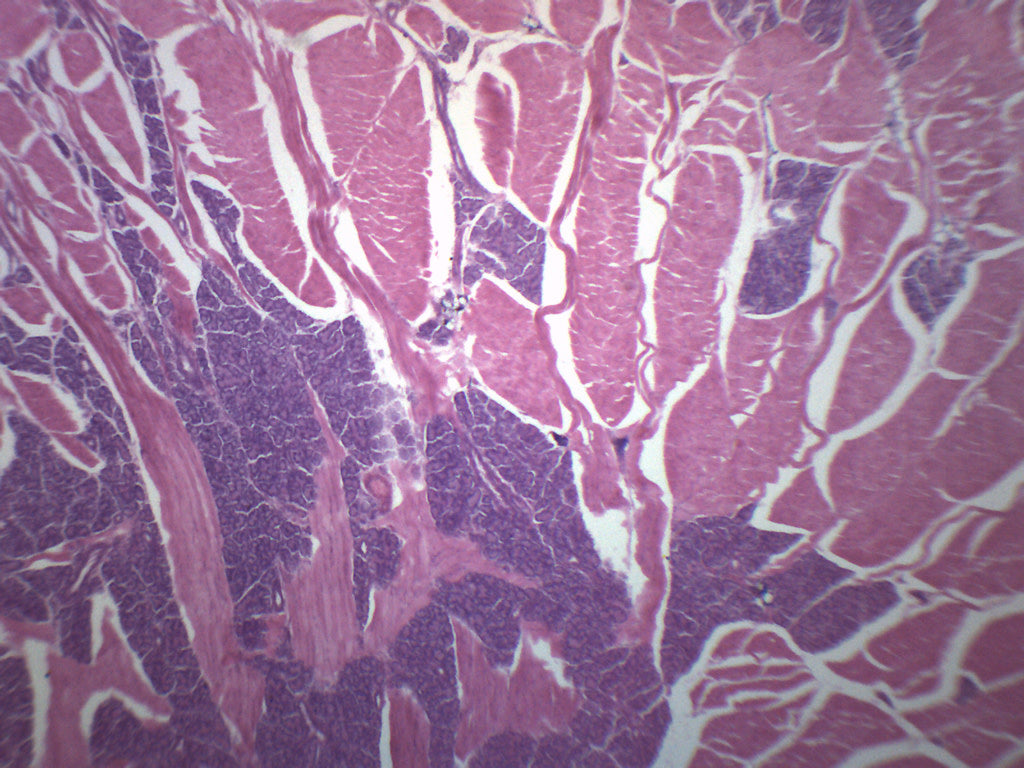This is a detailed and intricate image of a prepared microscopic slide showcasing the foliate papillae of a tongue. The photo reveals vertical columns in shades of pink interspersed with dark navy or blue, all bordered with white. As the view delves deeper into the tissue, the colors transition to a more complex interplay of navy and blue hues with gray speckles. The whole image has a marbled, abstract appearance with swirling patterns of dark and hot pinks, purples, and pronounced white streaks, almost resembling a mix of marbled meat. The unique combination of reds, whites, and other vivid colors creates a visually striking and scientifically valuable representation of the tongue's papillae structure.